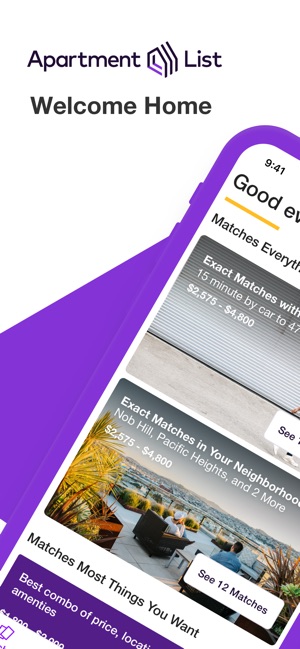The image features a promotional graphic with a white background. At the top, it displays the words "Apartment List - Welcome Home" in prominent font, set against the white backdrop. Below this, a purple line runs horizontally across the width of the image, intersecting with a purple smartphone graphic on the right side of the frame. The smartphone screen shows a time of 9:41, also against a white background. The screen displays the word "Good" in large text, underlined by an orange line, followed by partially visible text. 

Further down, the image provides housing options with specific characteristics: "Exact matches: Every TH" and includes details in a gray box specifying distances as "15 minutes by car to 4724." Price ranges for apartments are listed as "$2,575 to $4,800." 

There is a text box with the word "Boo," below which it reiterates "Exact matches" and lists neighborhood choices like "Nob Hill" and "Pacific Heights," with pricing again noted at "$2,575 to $4,800" and indicating "12 matches." Additional text at the bottom reads "Matches most things you want - Best combo of price, location, and amenities."